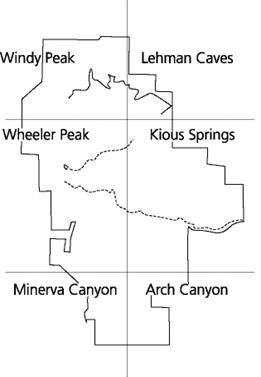This is a black and white, hand-drawn map on a white piece of paper, rendered in black ink. The map represents a square area divided into three sections by a central vertical line intersected by two horizontal lines. It identifies several locations, with labels in each section: Windy Peak in the top left, Lehman Caves in the top right, Wheeler Peak below Windy Peak, Kyle Springs below Lehman Caves, Minerva Canyon in the bottom left, and Arch Canyon to the right of Minerva Canyon. This structured layout suggests the map could pertain to a local region, likely in the southwestern United States, such as Utah, Arizona, or New Mexico. The boundaries of the map appear very linear and manufactured, rather than following natural features like rivers or mountains, hinting at an administrative or county division.